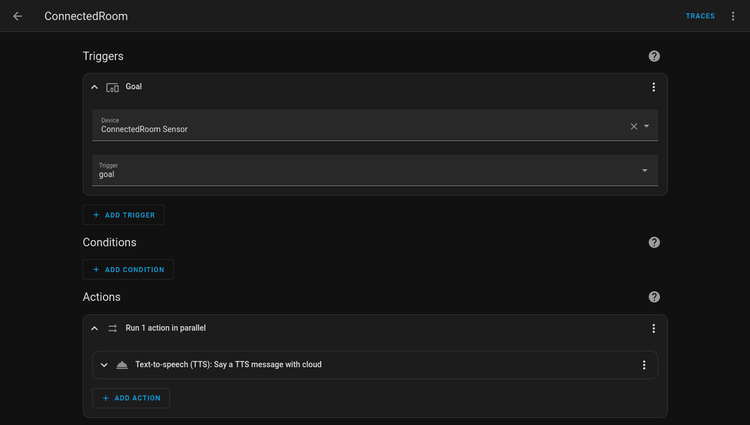This screen is a prototype for a potential website or app that categorizes various topics accessible within the platform. The background of the screen is black, complemented by dark gray tabs for a sleek and modern interface.

At the top of the screen, there is a navigation bar. On the left, it displays "Connected Room" accompanied by a leftward arrow symbol, while on the right, it reads "Traces" with three horizontal dots, suggesting additional options or a dropdown menu.

Below the navigation bar, the heading "Triggers?" in white font can be found, followed by several labeled sections. The first section lists "Goals" and "Connected Room Sensor and Trigger" under the context of defining a goal.

In subsequent sections, users have the ability to add specific elements, highlighted in blue font to indicate interactive buttons. The interface features an "Add Trigger" button denoted by a plus sign, enabling users to introduce new triggers into the system. Similarly, a section marked "Conditions?" also offers an "Add Condition" button with a blue plus sign, allowing the inclusion of new conditions.

Following the conditions section, an "Actions?" heading is present with the option to specify the execution as "Run One Action in Parallel." There are additional functionalities like "Text to Speech" (TTS) where users can program a message for the app to vocalize, indicated by an icon resembling a cloud. Lastly, another "Add Action" button, highlighted in blue text with a plus sign, is available for creating new actions within the system.

Overall, this detailed layout ensures users can efficiently navigate and manage triggers, conditions, and actions within the app.